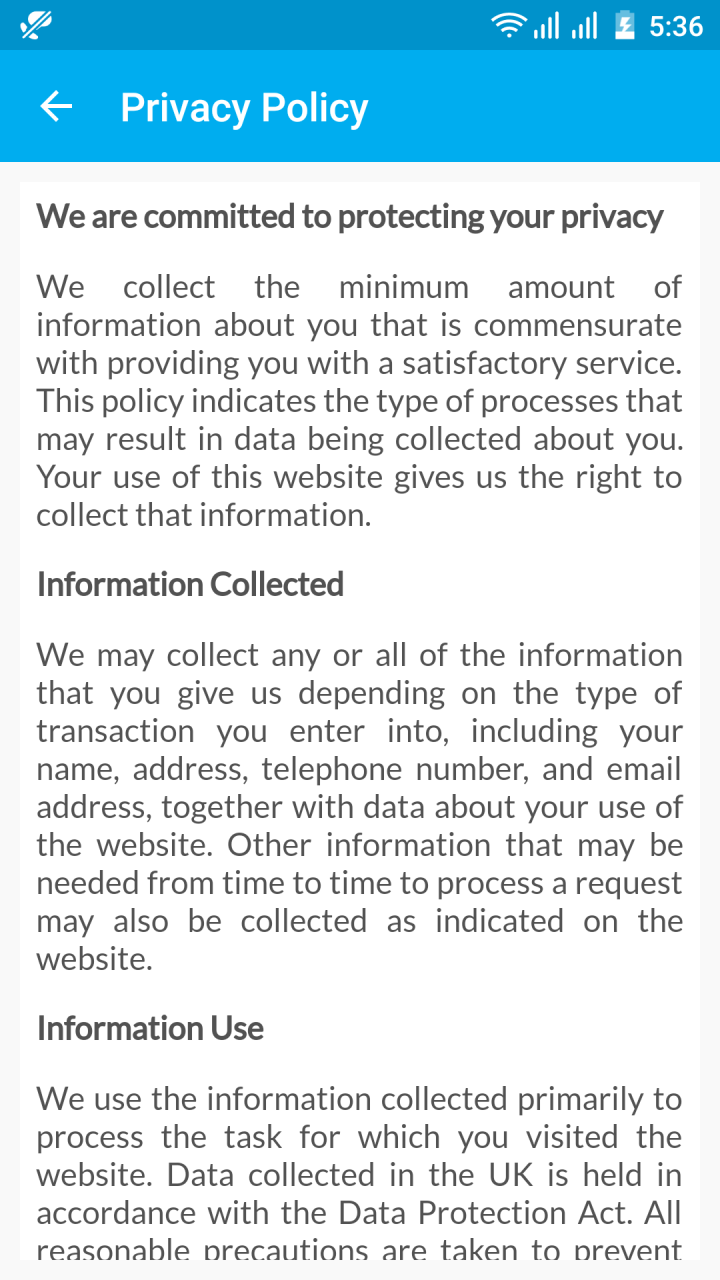A screenshot from an Android device displays a Privacy Policy document. The interface contains a light blue banner at the top, with a slightly darker blue banner above it. The document is presented on a white background, framed by a larger gray background. The Privacy Policy begins with the bold header "We are committed to protecting your privacy," followed by three paragraphs detailing how information is collected and used. The text is written in bold black font, making it clear and legible. In the top-right corner of the screen, icons for Wi-Fi, cellular signal, and a battery at approximately 25% capacity are visible, indicating the device needs charging. The time displayed is 5:36.